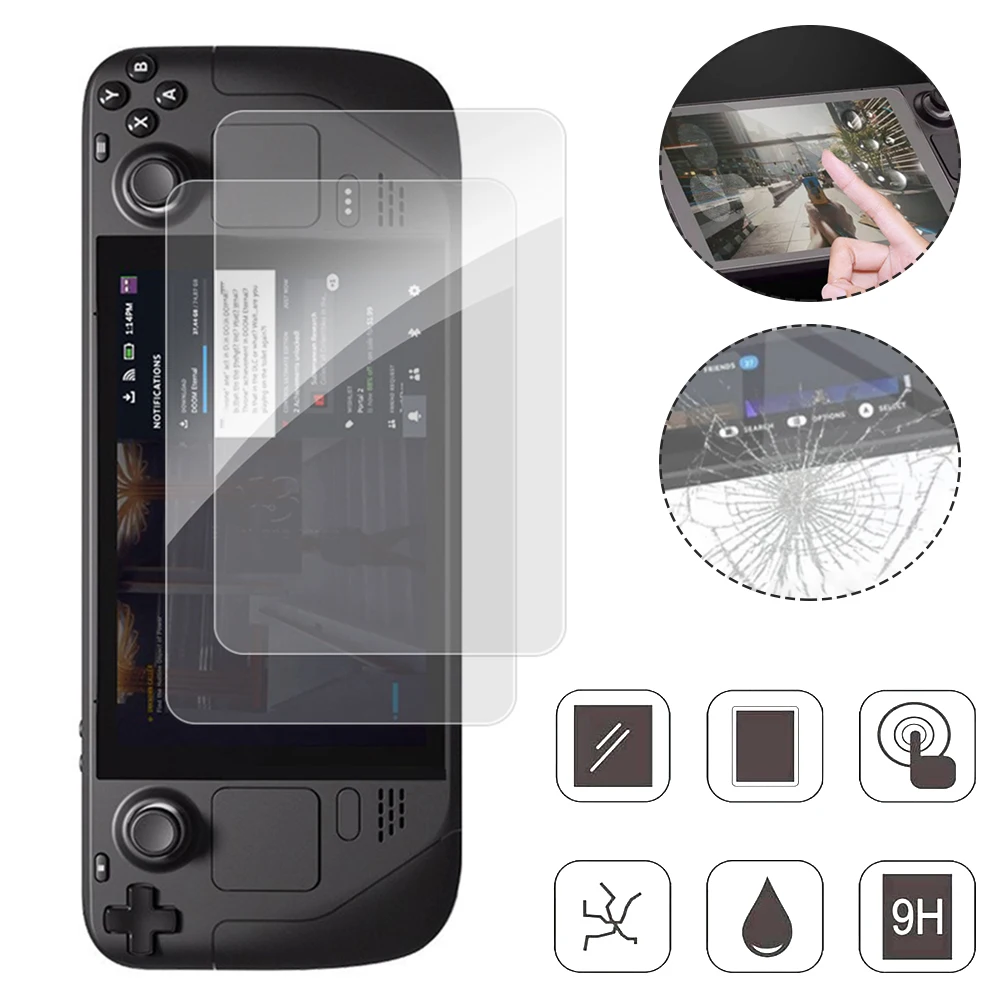The image is a detailed color illustration of a vertically positioned, all-black handheld gaming device, about the size of a cell phone. It features a small screen surrounded by various controls: a directional D-pad on the left, a joystick, and a set of four buttons labeled "A," "B," "X," and "Y" on the right, along with another joystick. White letters adorn the four buttons on the side of the device. The device is protected by two translucent screens hovering above it. To the right of the gaming device, there are two circular images: one depicting a finger touching the screen, and another illustrating a cracked screen. Below these circles are six smaller icons: a black square with two diagonal white lines, a solid black square, a circle with a finger pointing inside it, a stylized drawing of cracked glass, a single teardrop-shaped droplet, and a black square labeled with "9H" in white letters.